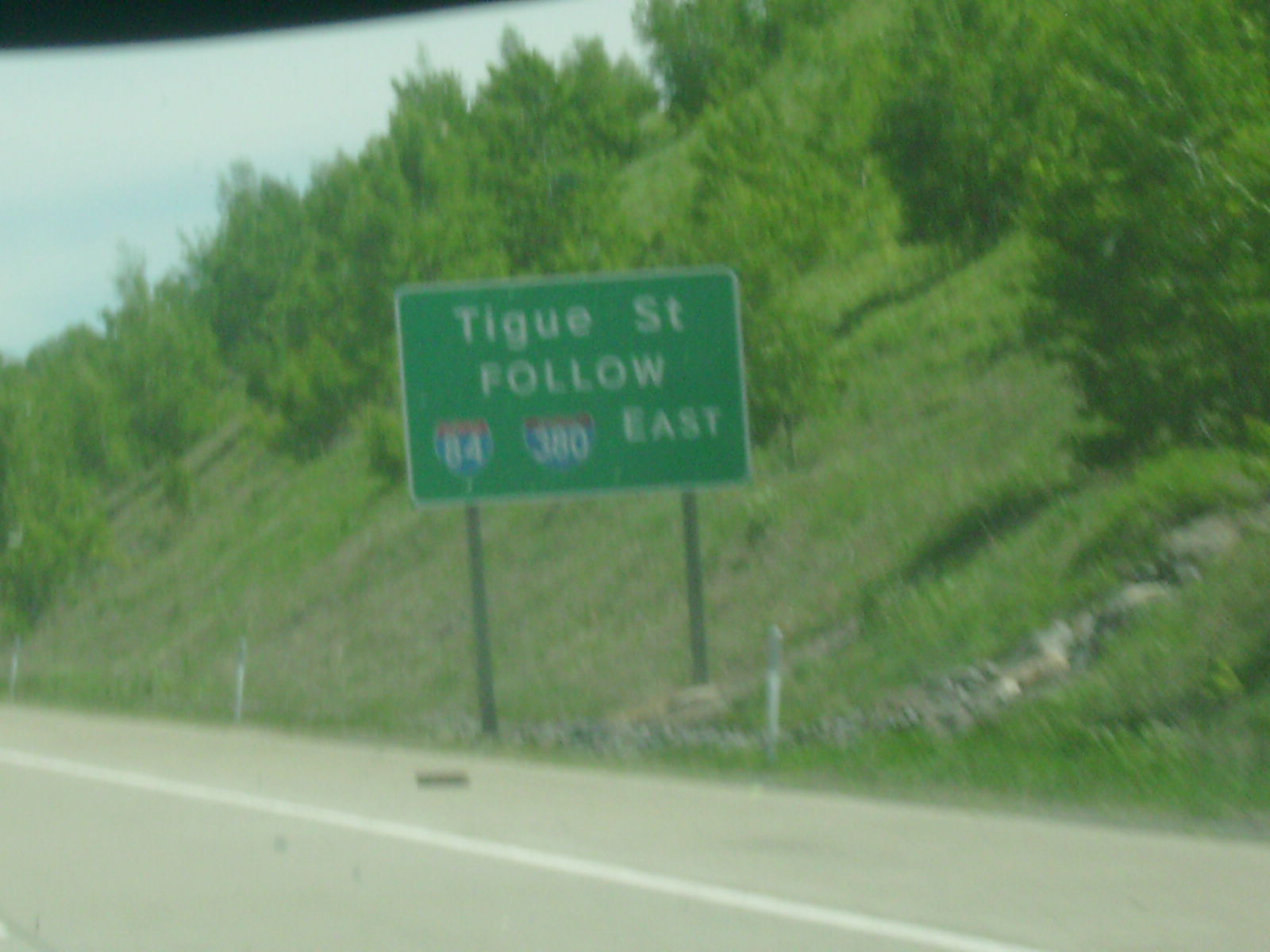This photograph captures a road scene taken from inside a moving vehicle, evident from the reflections on the glass and a glimpse of the door frame at the top. Dominating the image is a large, rectangular green road sign with a white reflective trim, held up by two black metal posts on the right side of the road. The sign, featuring white text, reads "TIGUE St, Follow 84, 380 East," with Interstates 84 and 380 indicated by blue and red numbers, respectively. The road below is marked with a white line, and on the side, there is a fence supported by white posts. In the background, a large hill covered with green trees and grass stretches up, giving the impression of a mountainous terrain, with parts of the stone foundation visible on the left.